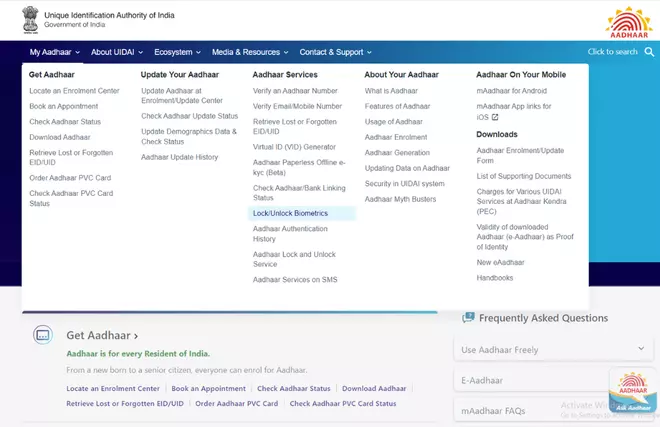In the top left corner of the image, there is a gray picture, adjacent to which you see the logo and text identifying the Unique Identification Authority of India (UIDAI). Below this, the text "Government of India" is displayed with a blue square as its background.

To the far upper right corner, there is an image resembling the top portion of a sun with short yellow rays and curved red lines within a white square.

At the top of the white square, black text horizontally lists several options: "Get AADHAAR," "Update Services," "About," and "On Your Mobile." Below this row is a clickable "Downloads" button.

In the center of the image, approximately halfway down, there is a blue rectangle with blue text reading "Lock/Unlock Biometrics." Additionally, in the bottom right corner, there is an option for "Frequently Asked Questions."